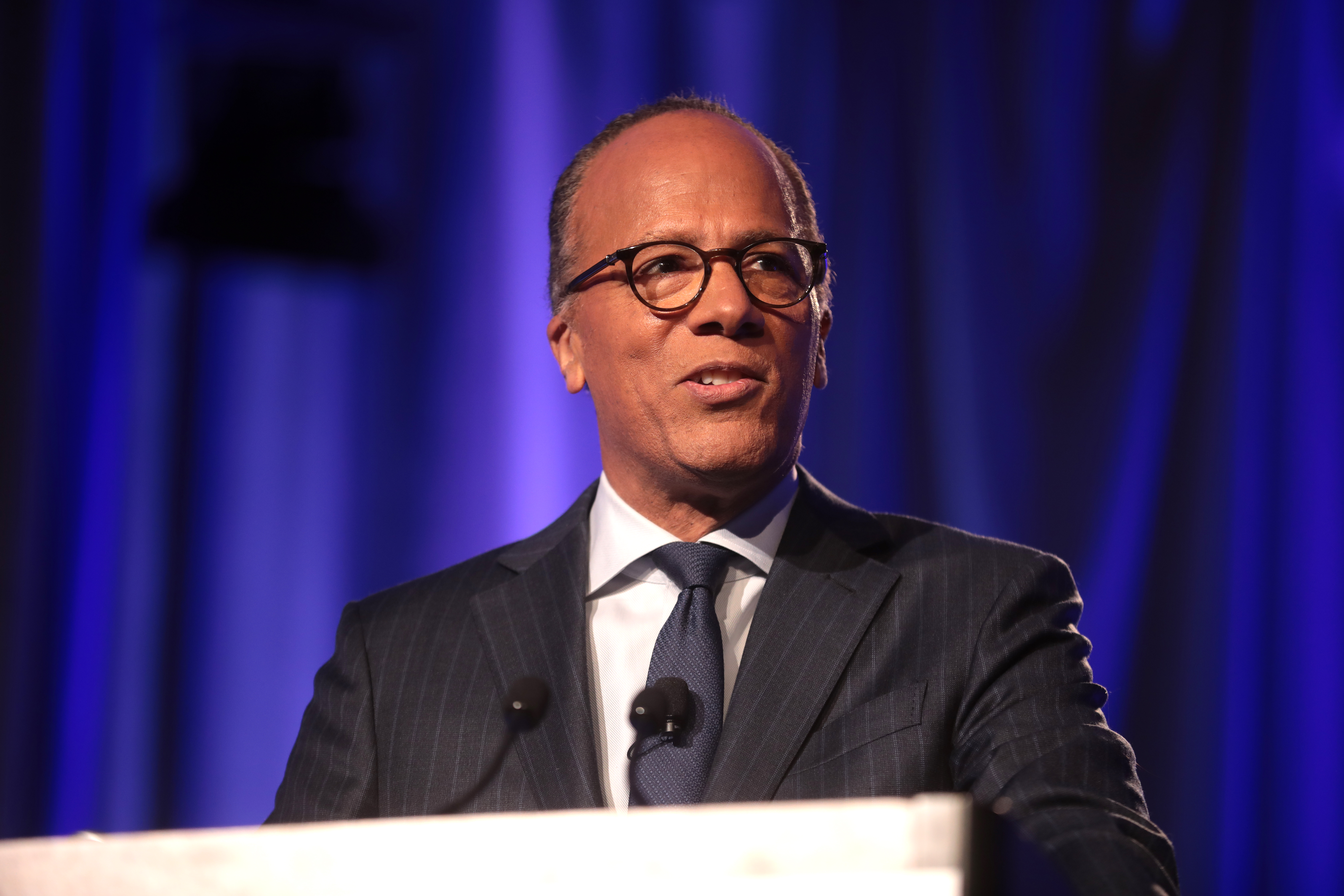The image features NBC News anchor Lester Holt standing at a podium. Holt, a Black man with a dark complexion, is dressed in a dark gray pinstriped suit with a dark blue tie and a white dress shirt. His outfit is complemented by large, round black-framed glasses. He is addressing a group, speaking into two thin-profile black microphones positioned on the podium in front of him, as well as a lapel mic clipped to his tie. His head is slightly tilted to the right with his mouth partially open, showing some of his teeth, indicating that he is in mid-speech. The podium is only partially visible at the bottom edge of the image. The background is blurred, with a mix of royal blue and purple shades, suggesting heavy drapery with vertical pleats. There is also an indistinct black shape in the upper left corner, likely part of the out-of-focus backdrop.